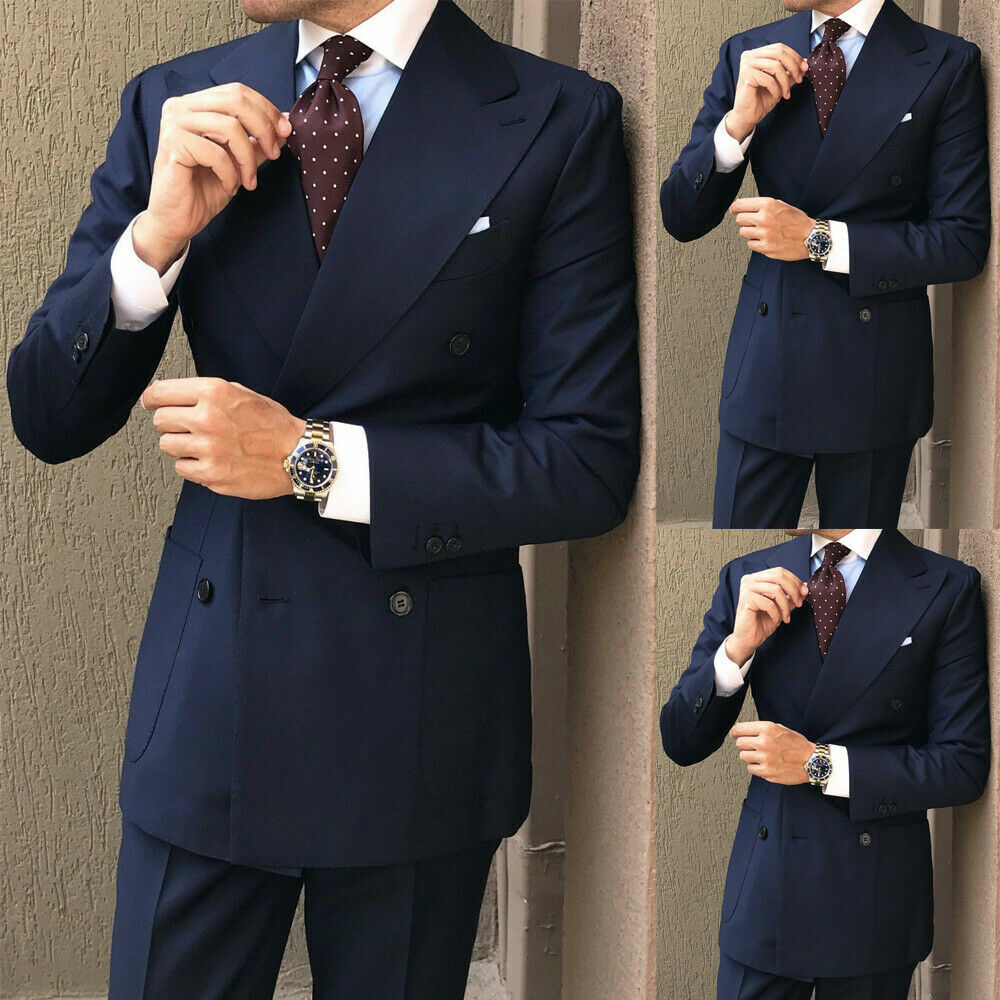The image features a collage of three identical pictures of a pale-skinned man in a well-tailored, navy blue double-breasted suit on a light tan wooden background. The larger picture on the left side shows the man from his chin to mid-thigh, while two smaller, identical images are stacked on the right. The suit jacket has four black buttons and two buttons on each cuff. He is wearing a white dress shirt and a maroon tie with white polka dots. His left hand is adjusting the tie, while his right hand, adorned with a silver watch featuring a dark face, is by his side. A subtle touch of a white pocket square peeks out from his jacket pocket, completing the sophisticated look.